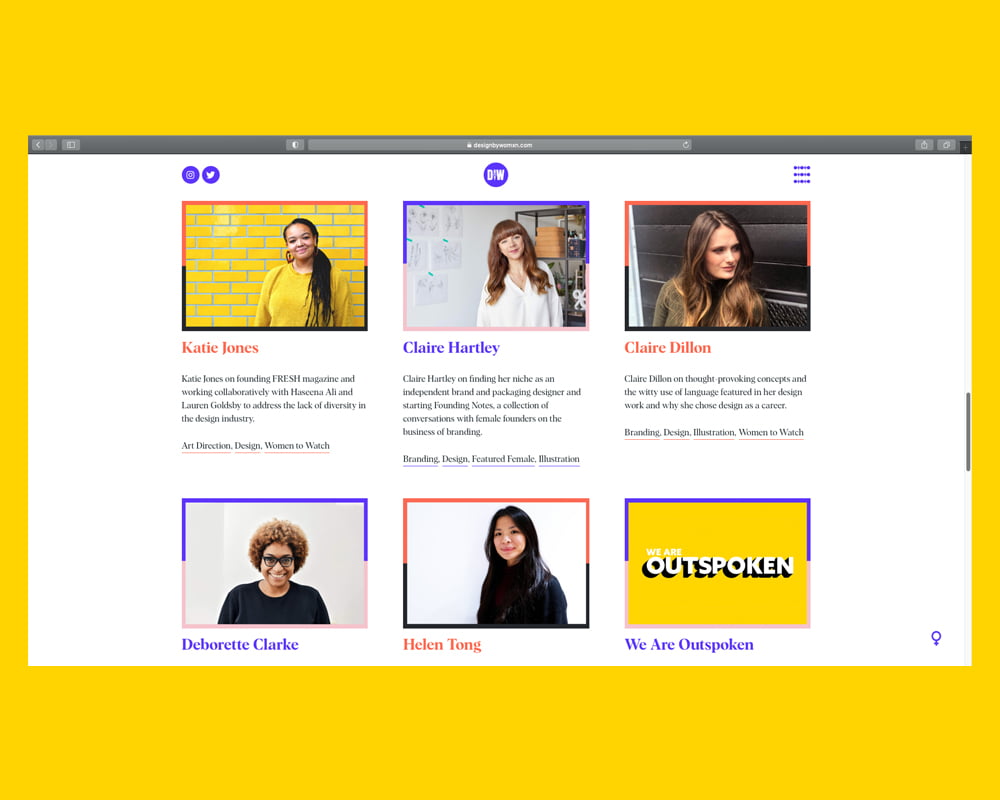The image depicts a website whose URL is indiscernible due to the small font size. The site's logo appears to be "DIW." The webpage features photographs of various women arranged in a grid format.

- **Top Left:** Katie Jones, a woman with long, dark hair, wearing a yellow shirt, stands in front of a backdrop of yellow bricks.
- **Middle:** Claire Hartley has red hair and is dressed in a white shirt. She is positioned to the right of Katie.
- **Top Right:** Claire Dillon, with long brown hair and a dark brown shirt, is also featured. 

In the row below:
- **Bottom Left:** Deborahette Clark, a woman with an orange afro and a black shirt.
- **Middle:** Helen Tong, who looks Asian, has dark brown, almost black hair, and is also wearing a black shirt.

On the far right of the grid, there is a yellow box with a text overlay stating "We Are Outspoken." The box has a blue or purplish edge along the top and a bit on the side. The entire webpage has a yellow background, creating a cohesive visual theme.